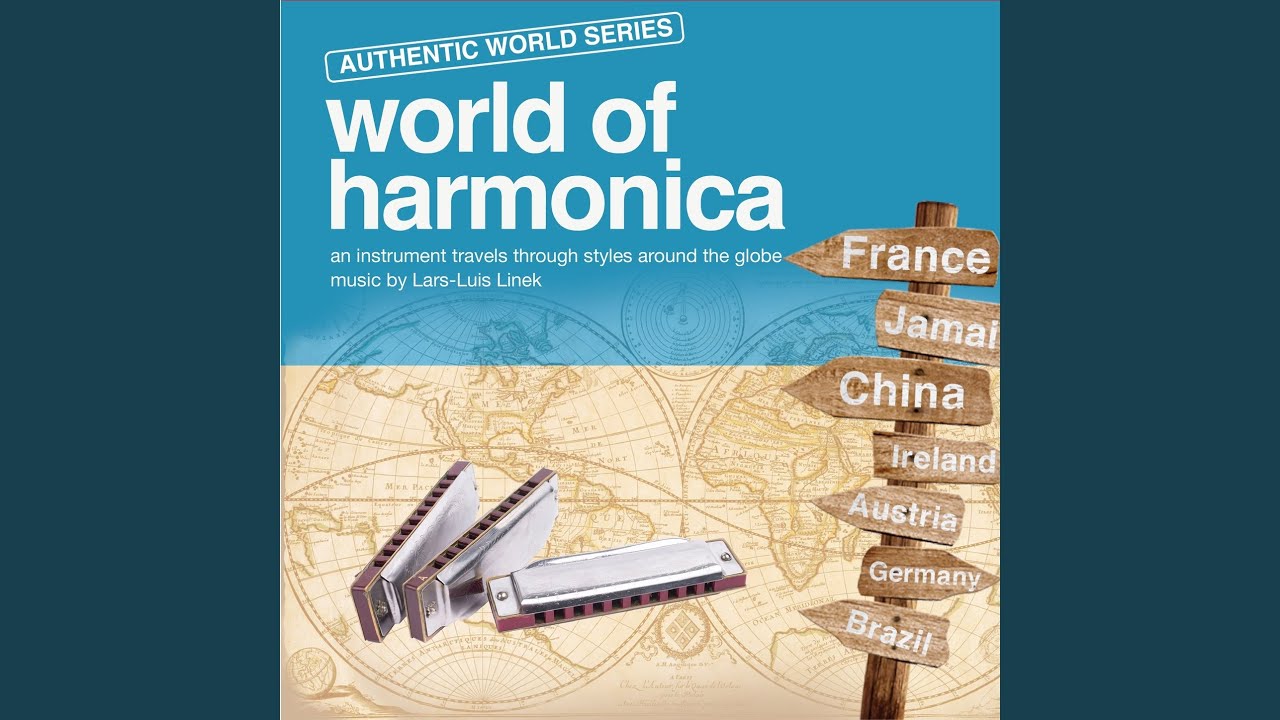The image is an album cover or advertisement titled "Authentic World Series: World of Harmonica, an Instrument Travels Through Styles Around the Globe" with music by Lars-Lewis Linek. The design uses a top block in a sky blue shade and a bottom block in a beige, off-white color, featuring an ancient, muted map of the world as the major background element. Prominently displayed in the center are three harmonicas, two standing on their sides and one lying flat. On the right side, there is an old-school wooden post with individual directional signs pointing to various destinations: France, Jamaica, China, Ireland, Austria, Germany, and Brazil. Each destination is labeled in white text on the wooden boards, contributing to the global theme of the cover.